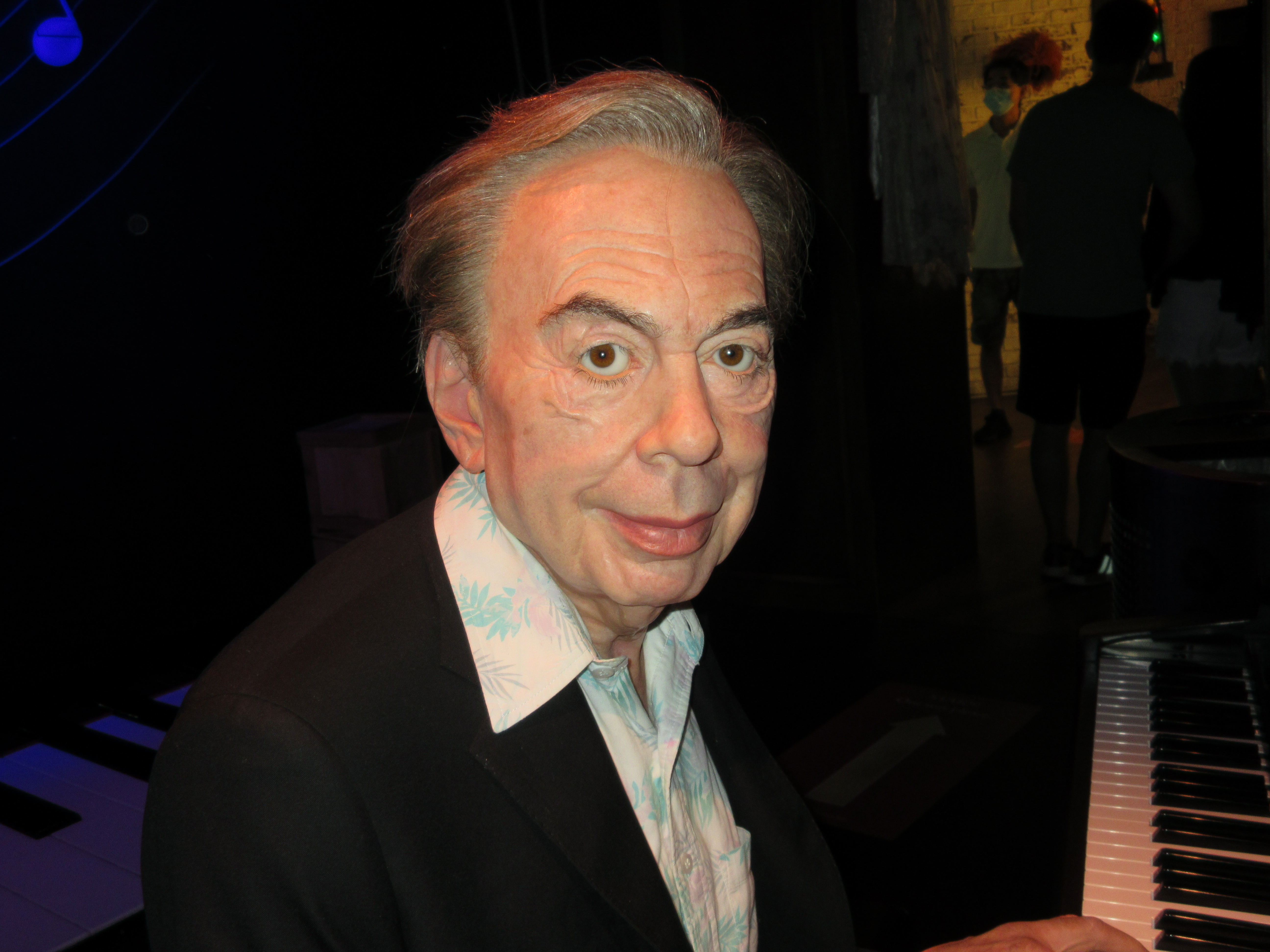The image features an older man, possibly in his 80s, who resembles Andrew Lloyd Webber. He is seated at a piano, with one hand resting on the keys, indicating that he is playing. He is dressed in a black jacket and a white button-down shirt, with the top button open at the neck. His face, which appears to have undergone some plastic surgery, shows slight droopiness and wispy gray hair brushed back from his forehead. His expression is a closed-mouth smile, and he is glancing directly at the camera while his body is turned to the right. The background of the image is predominantly dark, except for a blue light illuminating the top left-hand corner. In the distance, several people can be seen, some standing near what appears to be a doorway in the top right-hand corner, where additional light is seeping in. There also seems to be another keyboard visible in the bottom left behind him. The overall composition of the photo is horizontal and slightly rectangular.